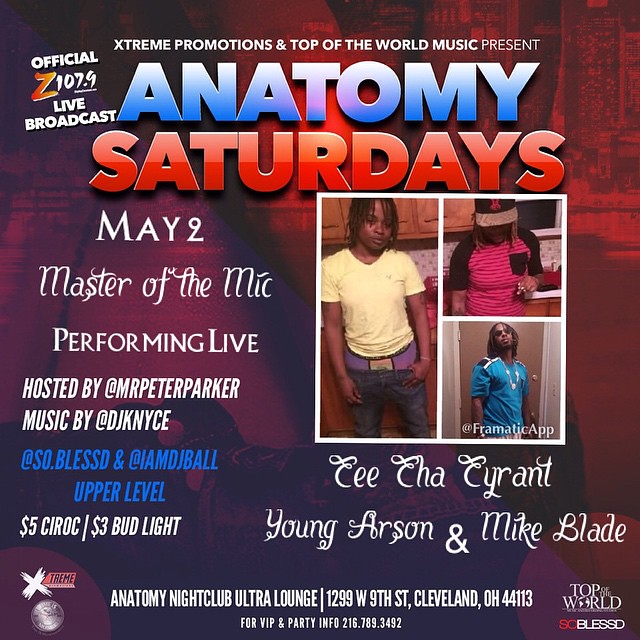This promotional poster is for a live musical performance titled "Anatomy Saturdays," presented by Extreme Promotions and Top of the World Music, with an official Z 107.9 live broadcast. The event highlights "Master of the Mic" performing live on May 2nd, hosted by Mr. Peter Parker. Music will be provided by DJ Knyce, DJ So.Blessed, and DJ Ball on the upper level. In bold blue letters, "ANATOMY" is prominently displayed, with "Saturdays" beneath it in red.

Down the left side, details include $5 Ciroc and $3 Bud Light specials. On the right side, there’s a montage featuring three images of the same black man with braided hair, wearing a yellow t-shirt, possibly taken in a kitchen setting. Below this montage, the names Cheat Tha Tyrant, Young Arson, and Mike Bleed are listed. At the bottom, the venue is specified as Anatomy Nightclub Ultra Lounge, located at 1299 West 9th Street, Cleveland, Ohio.